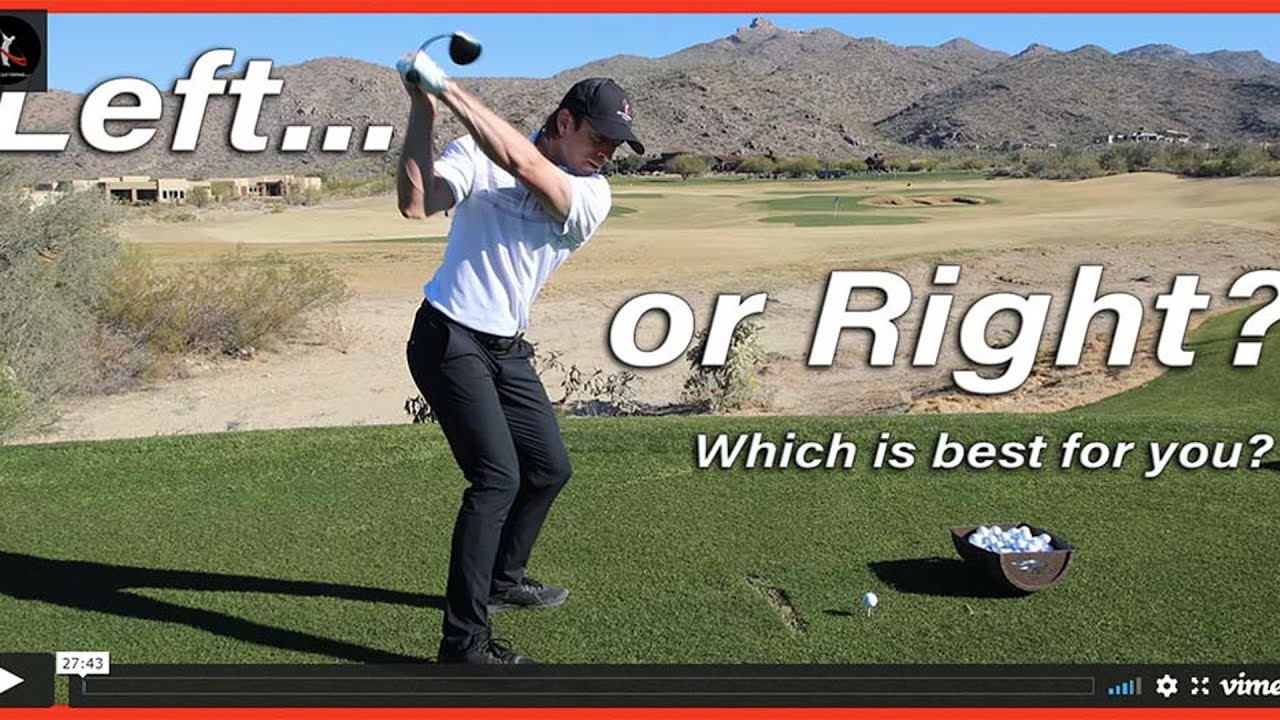This image is a screenshot of a Vimeo video paused at 27:43, showing a golfer preparing to take a swing on a desert-like golf course. It features a light-skinned male golfer in a white shirt, black pants, black shoes, and a black cap, concentrating intensely with his arms swung back and holding a golf club. He stands on green, smooth turf with a single white golf ball on a tee and a basket of golf balls nearby. The background includes sandy, arid land with mountains in the distance and some structures to the left. The screen capture has a horizontal red stripe at the top and bottom, blue volume marks, a settings icon, and the Vimeo logo at the bottom right. Overlay text reads, "left... or right? Which is best for you?"